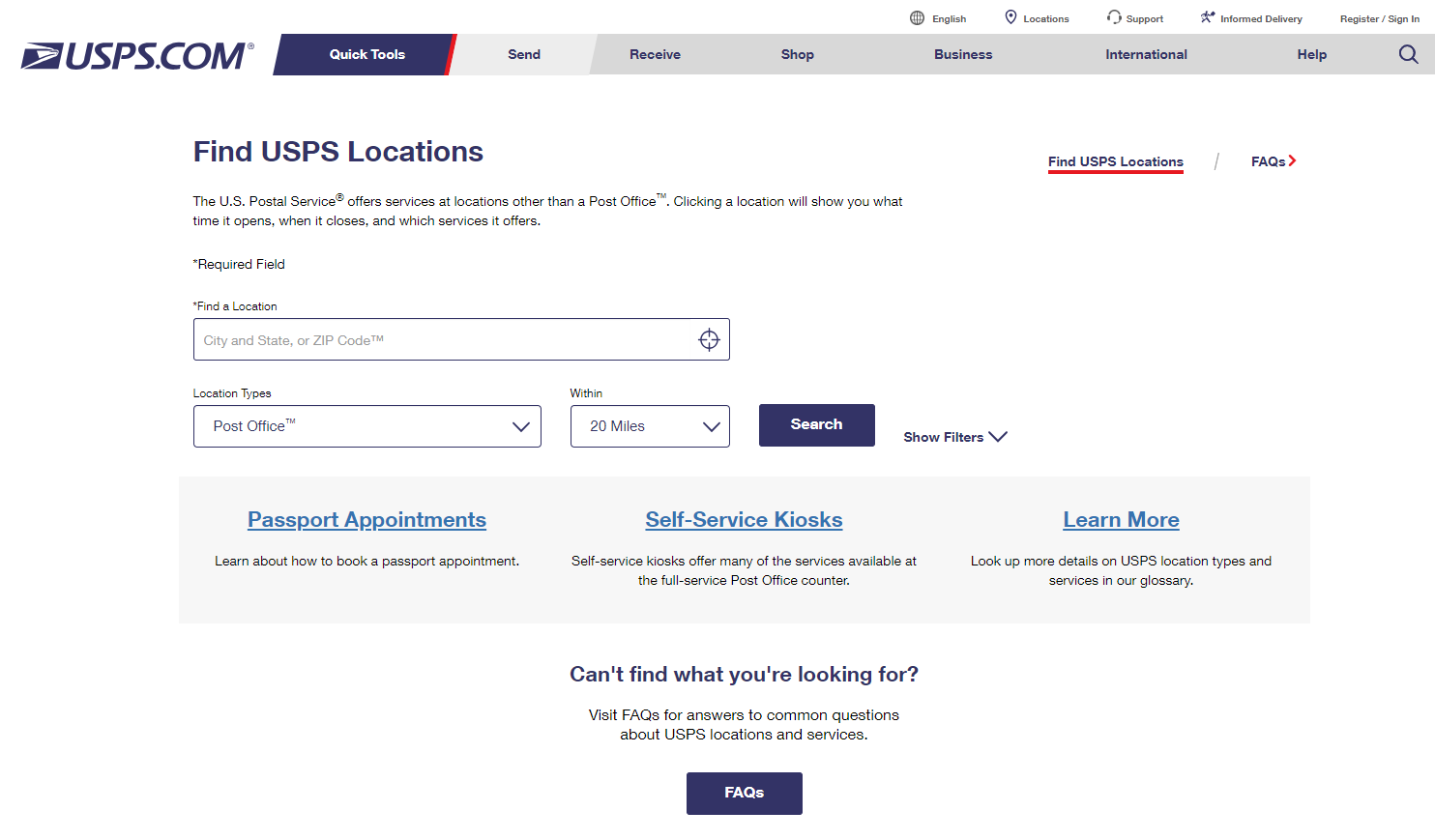This screenshot of a webpage from USPS.com captures a comprehensive view of their online interface, revealing essential navigational elements and functionality relevant to users seeking postal services. 

In the upper left corner, the recognizable USPS.com logo is prominently displayed. Adjacent to it, there is a horizontally aligned menu bar featuring the options: Quick Tools, Send, Receive, Shop, Business, International, and Help, along with a search icon. Notably, the "Quick Tools" tab is highlighted with a blue background and white text, whereas the remaining tabs are presented with a grey background and blue text, with the "Send" tab in a slightly lighter grey.

On the top right, the webpage offers features such as language selection (defaulting to English), location access, support options, and an "Informed Delivery" link, alongside a register/sign-in section.

Centrally beneath the main navigation, the page provides a primary feature to "Find USPS Locations," prominently presented with bold blue text. Below, an informative text advises users that the U.S. Postal Service offers various services and locations beyond traditional post offices. By clicking the location option, users can discover operational hours, closing times, and available services, with required fields marked by an asterisk. Users can search by entering a city, state, or ZIP code, and initiate the search via a dark blue button labeled with white text.

Further customization is available through dropdown lists: one to select the type of location (defaulted to "Post Office") and another to define the search radius (with "20 miles" selected). Additionally, a filter option can be accessed through a downward-pointing arrow. To the right, there is an underlined, clickable red link labeled "Find USPS Locations" and a related FAQ section marked by a red arrow.

Below, the webpage is divided into three light blue sections, each offering specific information:
1. **Passport Appointments:** Guidance on scheduling appointments for passport services.
2. **Self-Service Kiosks:** An explanation of the services available at self-service kiosks, comparable to those at a full-service post office.
3. **Counter and Glossary:** Details on different USPS location types and services, accessible through a glossary.

At the bottom of these sections, assistance is offered for users unable to find what they need, directing them to a comprehensive FAQ page through a dark blue button labeled "FAQs" in white text.